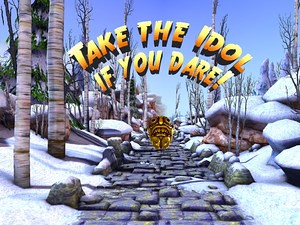A vibrant game interface is depicted in a square image likely found on a mobile phone. At the center top, bold yellow text transitions to orange at the bottom, declaring "Take the idol if you dare!" Below this text lies a golden idol resting on a cobblestone gray path that winds into the distance. To the right of the path, snow-covered rocks are piled high, while to the left, more snow decorates the landscape alongside what appear to be the gray trunks of palm trees. The trees lining the road are bare, their leafless branches reaching upwards. The sky overhead features a gradient from dark blue at the top to light blue near the horizon. The image strikes a balance of colors, including various shades of blue, white, touches of green, yellow, and orange for the text, and gold for the idol. The scene sets the stage for an adventurous gaming experience centered around capturing the coveted idol.